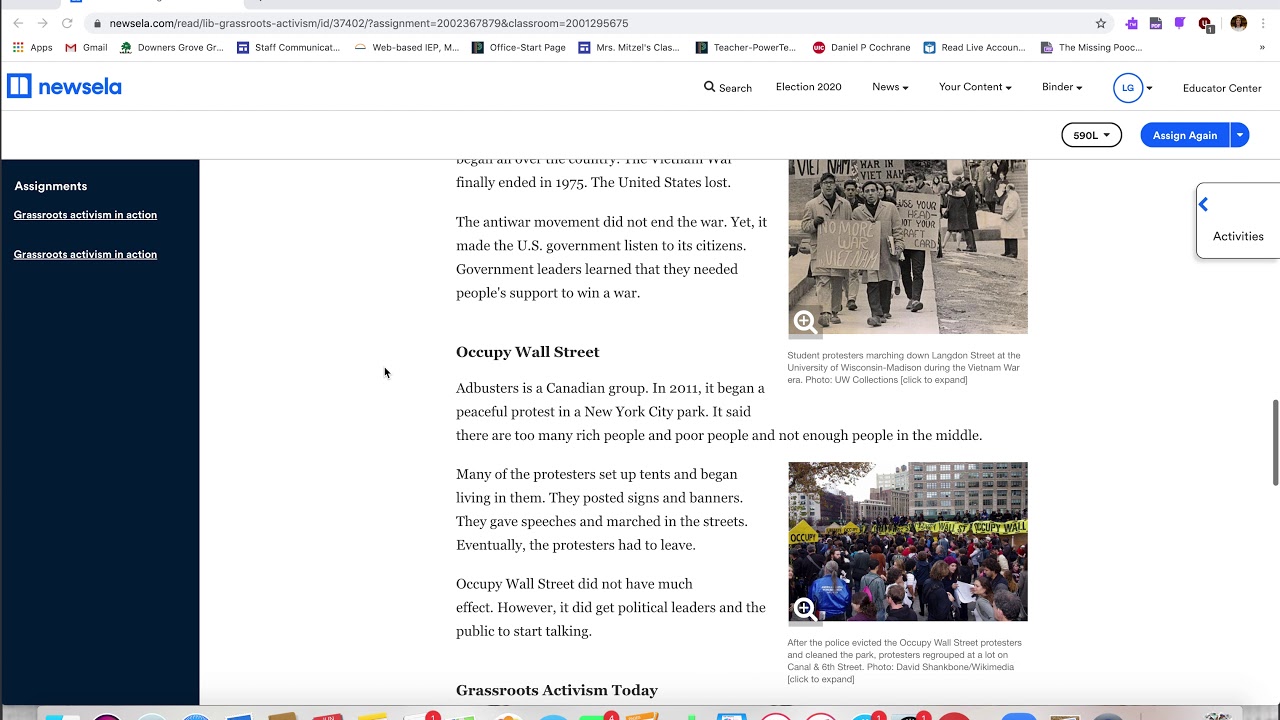This screenshot of the Noosala platform showcases a blue-themed interface with multiple features visible on the screen. Prominently displayed are tabs labeled "Search," "Election 2020," "News," "Your Content," "Finder," "Educator," and "Center." On the left side of the screen, there's a section marked "Assignments," although the specific words are too small to decipher clearly. However, there are notable mentions of "Activism and Action," likely repeating twice, and each word presumably starts with a G.

The screenshot also includes the beginning of an article. The article discusses the impact of the anti-war movement, noting that while the movement did not end the war, it succeeded in making the U.S. government more receptive to its citizens. It highlights that government leaders realized the necessity of public support to win a war. Another section of the article covers the "Occupy Wall Street" movement. It mentions that Adbusters, a campaign group, initiated a peaceful protest in a New York City park in 2011 and provides further information on this topic.